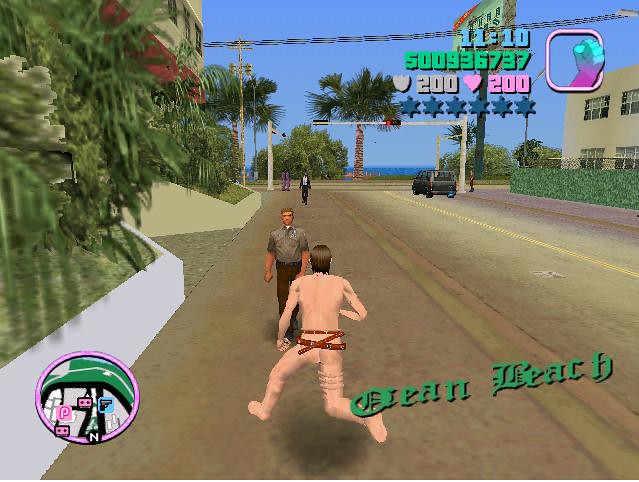This screenshot from a video game captures a vibrant urban scene. Dominating the foreground are two cartoonish characters; one appears to be a nearly-naked runner, wearing only a belt, seemingly in the midst of an escape, while an approaching police officer closes in on them. The action unfolds on a road bordered by a spacious sidewalk. Adjacent to the sidewalk are large white planter boxes topped with lush greenery, adding a touch of nature to the cityscape. A descending road bisects the scene, drawing the eye toward the background where picturesque palm trees stand tall against the serene backdrop of the ocean. A stoplight marks the intersection further down the street, where a few more animated figures can be seen. The top right corner of the screen prominently displays the location as "Ocean Beach," framing the entire composition within a bustling, coastal environment.